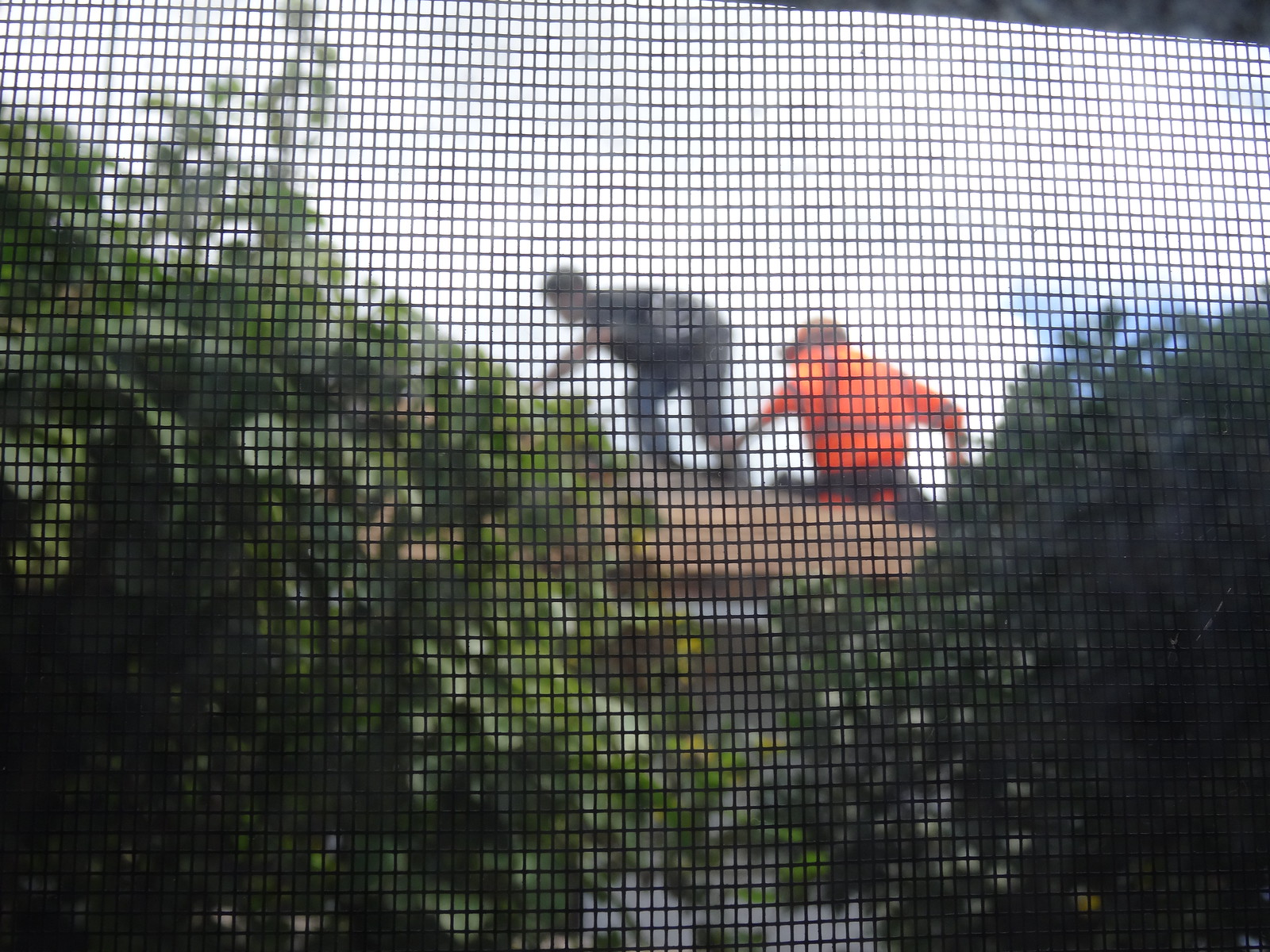This photo, taken through a screen window or door, features a grid of black vertical and horizontal lines that create a pixelated effect. The image is predominantly blurry due to the screen and distance. It shows a couple of men working on the roof of a house, partially visible between two green trees or shrubs on the left and right sides. The men are fairly indistinct but can be made out by their attire: the man on the right is wearing a neon orange shirt, resembling a construction safety shirt, potentially with silver or gray stripes, and appears to be sitting or crouching. The man to his left, wearing a black shirt, looks to be in the process of climbing or working on the sloped brown roof of what seems to be a white house. Overhead, the sky appears light blue. The view is captured from a home interior, peering through the mesh screen, creating a magnified effect on the screen pattern.